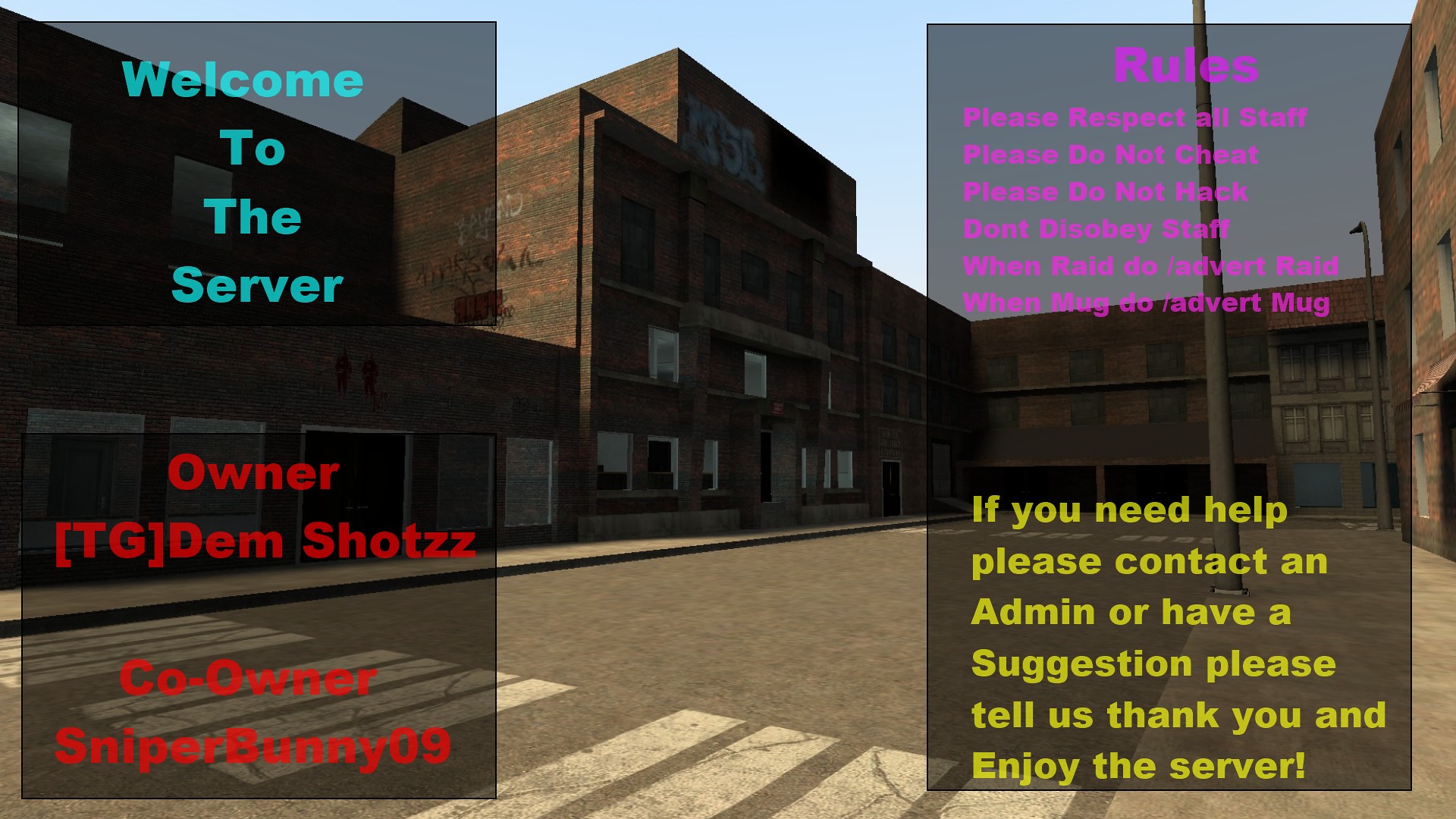The image depicts an outdoor setting, showcasing an empty road with a zebra crossing in the foreground, leading to a dead end marked by brown, apparently abandoned buildings in the background. The sky is visible above the buildings. Superimposed over this scene are two semi-transparent, grey rectangular text blocks. The left text block features a warm welcome in light blue text that reads, "Welcome to the server." Below this, in red text, it lists the server administrators: "Owner: TG Dem Shots" followed by "Co-Owner: SniperBunny09." On the right text block, the header "Rules" is written in purple. Beneath this, a series of directives are provided in purple text: "Please respect all staff. Please do not cheat. Please do not hack. Don't disobey staff. When raid, do /advert raid. When mug, do /advert mug." At the bottom, in yellow text, the box advises: "If you need help, please contact an admin or have a suggestion. Please tell us. Thank you and enjoy the server."